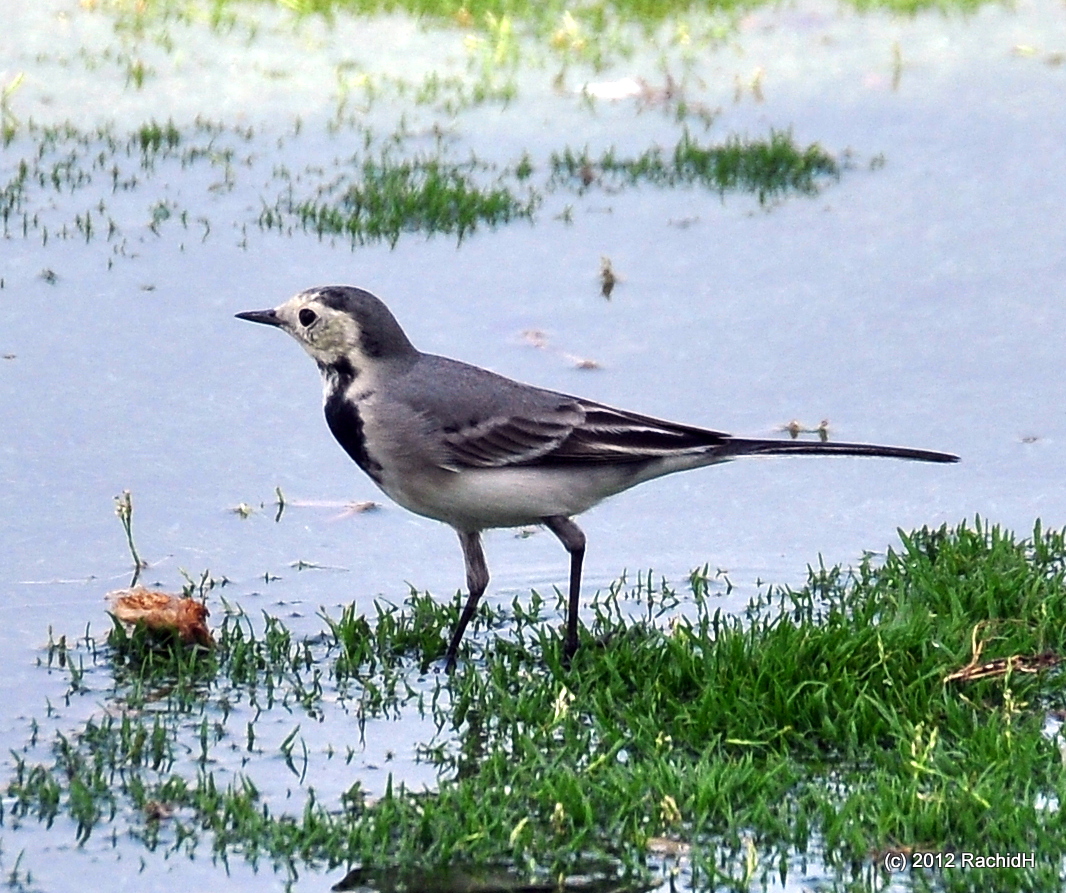The photograph captures an intricate scene of a marshland where a bird stands gracefully in the shallow water. The bird, likely an Oriole, is positioned centrally in the image, facing to the left. It boasts a striking plumage with a black chest, a whitish-gray underbelly, and wings that are medium dark gray with black striations at the tips. The bird's tail feathers are black, and it has a black beak and a distinctive black cap atop its mostly grayish-white face.

In the foreground, there's a ripple effect around the bird's thin legs, indicating its slight movement in the water. Surrounding the bird are tufts of green grass protruding from the water, giving the habitat a lush appearance. Scattered twigs and foliage float around, enhancing the natural ambiance of the scene. Besides the bird, noticeable is a small red flower and some brown object among the grass, adding a splash of color and texture.

In the background, the image transitions to more open water with sporadic patches of grass, leading to a denser grassy area towards the top. The bottom right corner of the photograph contains white lettering stating "Copyright 2012 RACHID H," marking the credit of the image author.